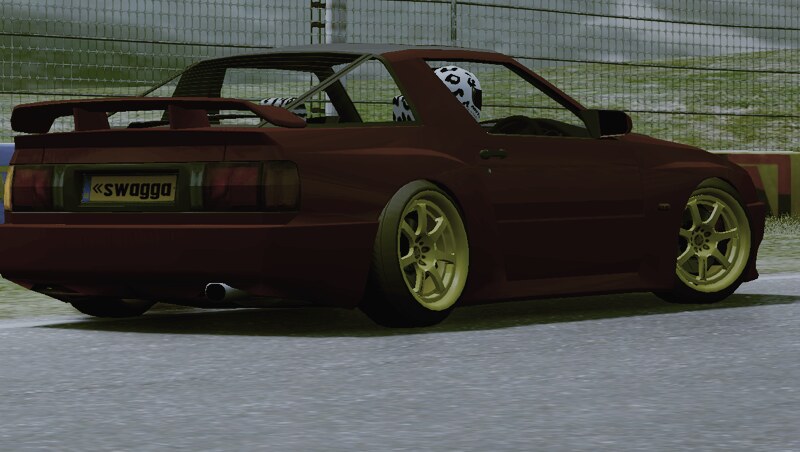This image appears to be a detailed 3D rendering or a screenshot from a video game, depicting a dark burgundy sports car on a racetrack. The car, which has a reddish-brown hue, features striking gold-silver rims and a noticeable scoop on the back trunk. An identifiable detail is the yellow-gold license plate with the bold black letters "SWAGGA." The vehicle has no roof, and the windows are rolled down, revealing occupants wearing white helmets with black splashes or leopard print designs. The racetrack is paved in gray, and in the background, there is a chain link fence attached to a short, reddish wall, providing a barrier to dry grass-covered hills. The scene is set under an overcast sky, adding to the overall realistic yet slightly unreal video game graphic quality.